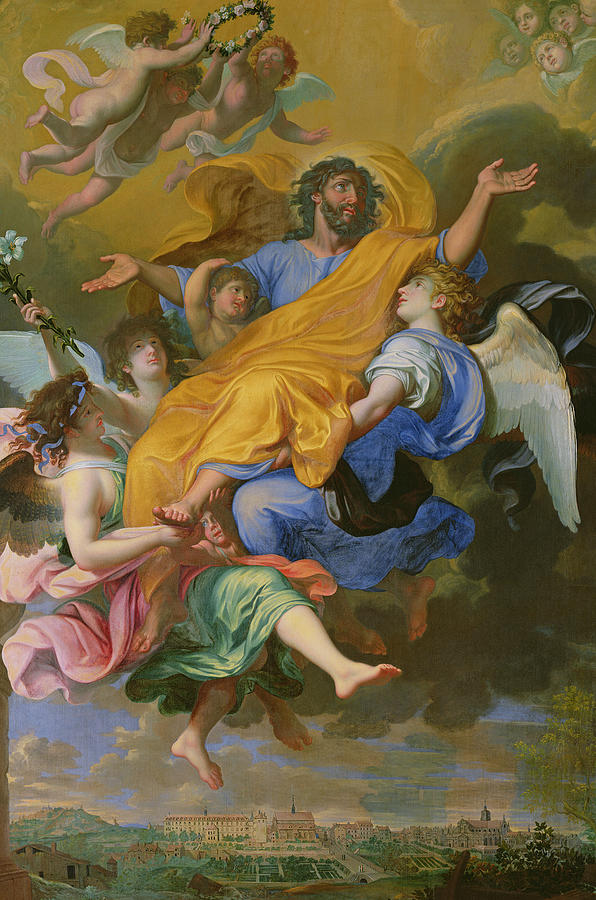This detailed painting, reminiscent of the style of Leonardo da Vinci or old Italian Masters, presents a central figure, likely Jesus, with flowing hair and a beard, dressed in a blue garment and adorned with a golden sash. His arms are extended outward, creating a sense of openness. Surrounding him are angels, some depicted as young, Cupid-like figures with curly hair and delicate wings. They appear to float mid-air, with several supporting Jesus from below. The angels are unclothed, save for some adorned in white ribbons and sashes, and they hold a wreath of green leaves and pink flowers. One angel clutches a green-stemmed flower with white petals. 

The background features a detailed cityscape or castle, enhancing the Renaissance feel with its deep, dark hues. The setting includes a sky filled with clouds, amplifying the ethereal atmosphere of the painting. Additional details include angels in various colored robes—yellow, green, pink, and blue—emphasizing the realism in their skin tones and textures. Toward the top right corner, a group of child-like angels huddled together and seemingly observing the scene add to the intricate composition. This evocative piece, likely showcased in a museum, captures a masterpiece that blends celestial elements with a serene terrestrial backdrop.